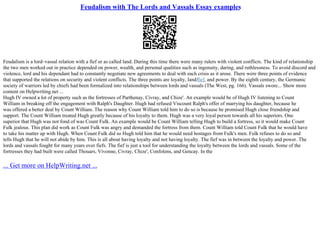The image features a printed document displayed on a white background. The main title, displayed prominently at the top in blue, reads "Feudalism with the Lords and Vassals Essay Examples." Directly beneath the title is a QR code, which is square-shaped and positioned centrally. The document also has two paragraphs of text below the QR code, but they are extremely small and out of focus, making them virtually unreadable. The first paragraph appears to discuss the dynamics of feudalism, mentioning terms like "thief," "land," "loyalty," "negotiations," "Lord," and "Germany," though much of it is indecipherable. The second paragraph seems to reference historical figures and events, including names like Hill IV, Count William, and Viscount Ralph, but again, the text is largely illegible.

At the very bottom of the document, there is another line of blue, hyperlinked text that reads, "get more on helpwriting.net." This likely indicates a website where additional essay-writing assistance can be found. Overall, the document seems to function as a tool for obtaining essay examples or writing help, possibly aimed at students looking to either get inspiration or "Cliff Notes"-style summaries for their own work.